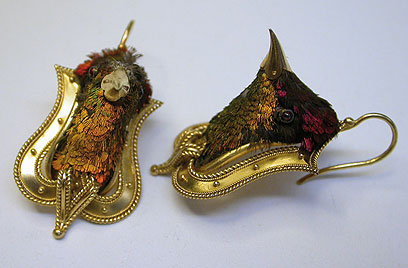This image showcases a pair of ancient-looking gold jewelry pieces, which appear to be earrings. Each earring features a highly ornate design, consisting of a central, multicolored bird head mounted on a horseshoe-shaped gold structure with a rope-like edge. The birds have iridescent plumage, with one displaying a mix of gold and purple hues with a golden beak, and the other exhibiting darker feathers with hints of red and orange. The jewelry pieces include thin gold wires, possibly designed to hang from the ear. The photo background is light blue, providing contrast to the intricate details and the vibrant colors of the bird heads.